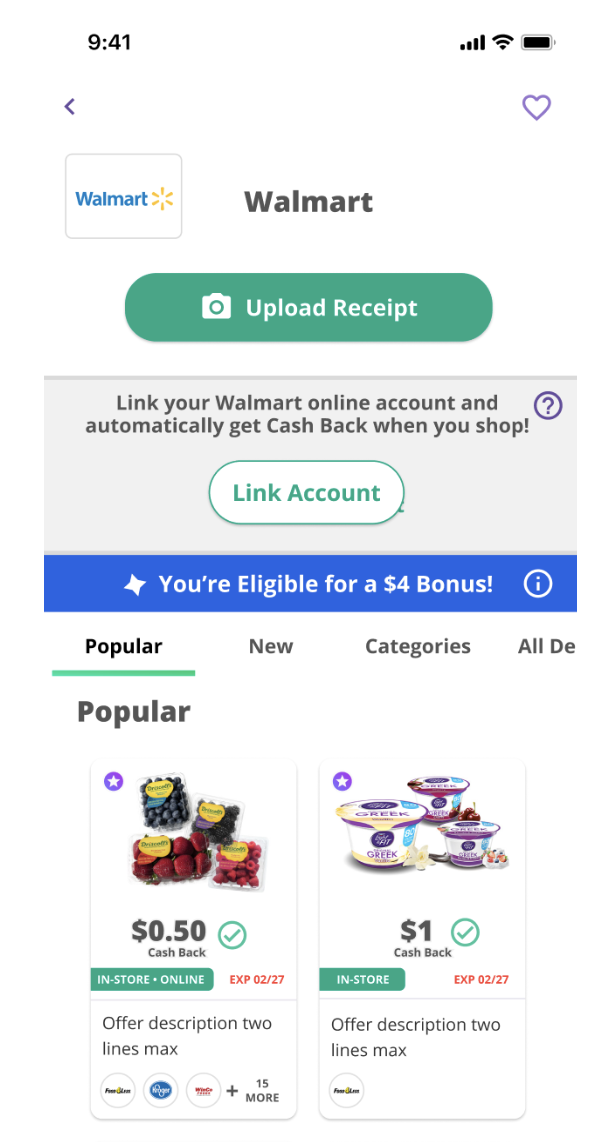The screenshot depicts a user interface from a mobile application with the following features:

- At the top, the phone status bar indicates it is 9:41 AM, with a full battery and full signal strength. It also displays a heart icon and a left stand icon.
- Below the status bar, the Walmart logo is prominently displayed within a rectangular box.
- Under the logo, there's a dark green oblong button featuring a camera icon, accompanied by the text "Upload Receipt."
- Situated below the green button is a gray box containing a prompt that reads: "Link your Walmart online account and automatically get cash back when you shop." A linked white button in the box says "Link Account."
- A blue tab underneath announces, "You're eligible for a $4 bonus."
- Following this, a navigation bar includes tabs labeled "Popular," "New," "Categories," and "All Deals." The "Popular" tab is selected, indicated by a green line beneath it.
- The main content area under the tabs is divided into two sections:
  - The left box displays "$0.50" and an offer description truncated to two lines.
  - The right box shows an image of yogurt with "$1" and a similarly truncated offer description.

This detailed visual captures the key elements of the app’s interface, outlining both its functionality and layout.